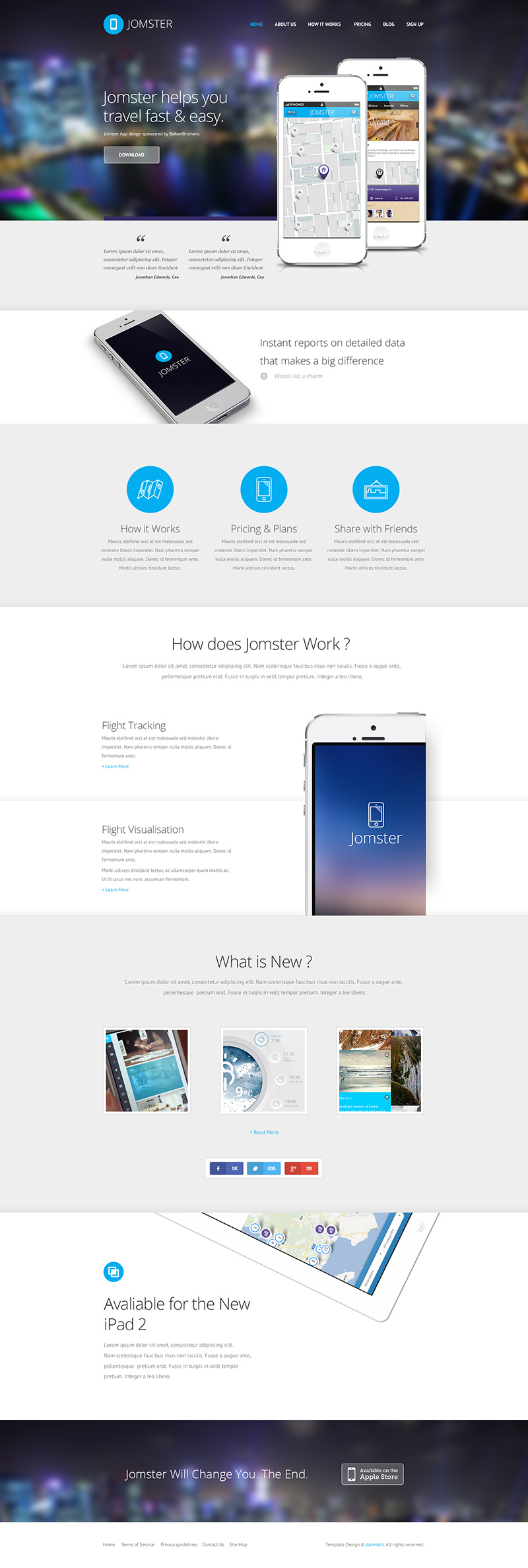**Screenshot of Jomster Web Page**

This image showcases a web page or smartphone app called Jomster, designed for flight tracking and visualization. The page features a vibrant, horizontally spanning multicolored banner at the top, displaying a spectrum of colors: black, purple, blue, white, yellow, and green. 

In the top-left corner of the banner, the word "JOMSTER" is prominently displayed in all capital letters. At the center of the banner, the tagline "JOMSTER helps you travel fast and easy" is proudly presented. To the right of this text, two overlapping images of tablets, both running the Jomster program, are depicted with the left tablet on top.

Beneath this banner, on the left side of the screen, a diagonal image of a cell phone is prominently featured. To the right of the cell phone, the text reads, "Instant reports on detailed data that makes a big difference." Below this, a series of blue, oval-shaped designs are arranged horizontally across the screen, each containing white drawings that are too small to discern in the screenshot provided.